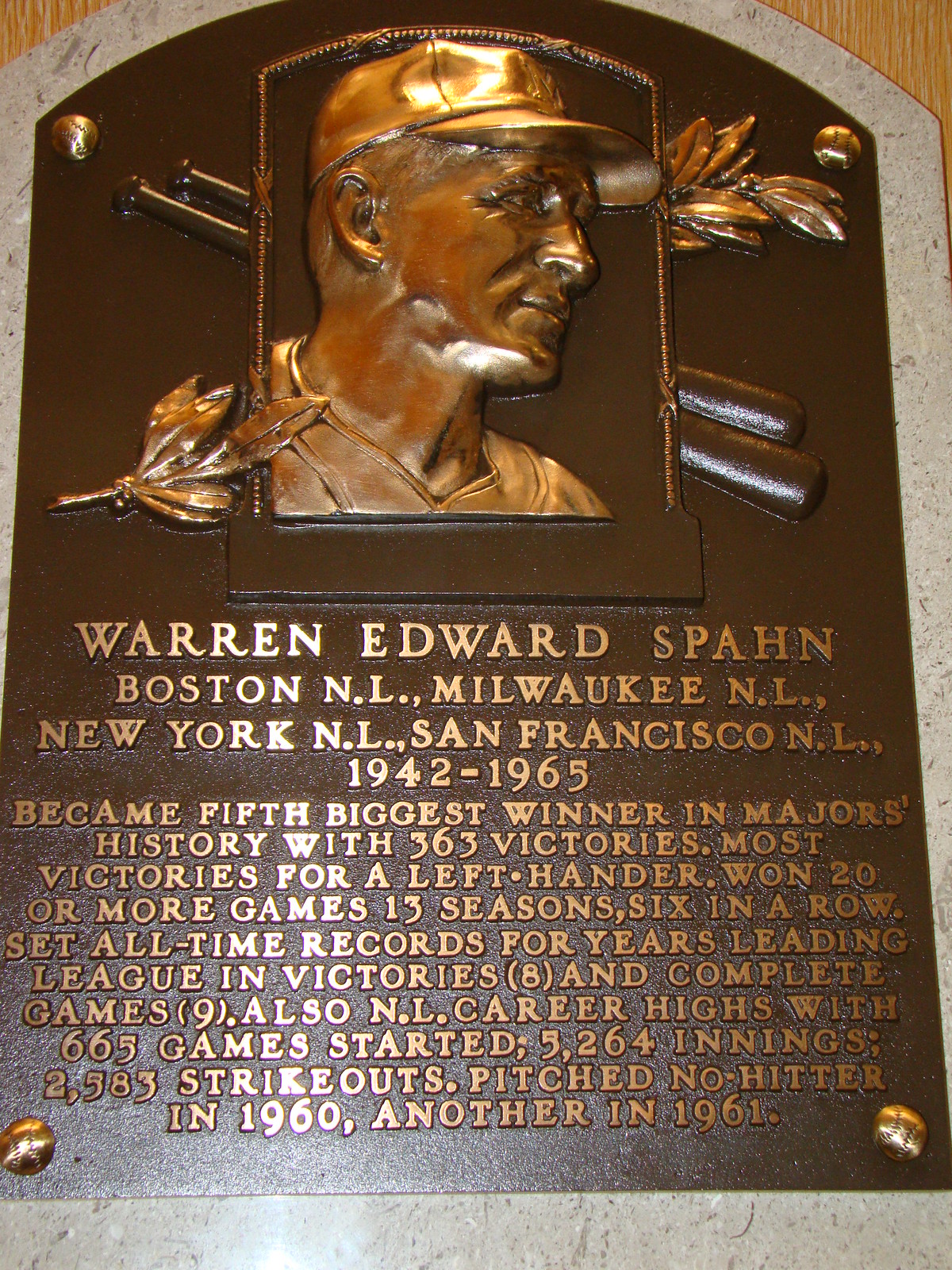The image showcases a bronze commemorative plaque dedicated to Warren Edward Spahn, notable baseball player for the Boston NL, Milwaukee NL, New York NL, and San Francisco NL from 1942 to 1965. The upper part of the plaque features a raised bronze relief of Spahn wearing a baseball cap and looking to the right. Behind him, there is an engraved outline of a baseball bat and decorative leaves. The plaque is predominantly dark bronze with gold lettering, featuring Spahn's remarkable achievements, including becoming the fifth biggest winner in major league history with 363 victories, most victories for a left-hander, and winning 20 or more games in 13 seasons, six consecutively. It also highlights his all-time records for leading the league in victories and complete games. Notably, he started 665 games, pitched 5,264 innings, struck out 2,583 batters, and threw no-hitters in 1960 and 1961. The edges of the plaque are bordered by a stone or marble frame and it's mounted on a wooden surface. Additionally, the nails fastening the plaque are shaped like baseballs, adding a unique touch to the piece.